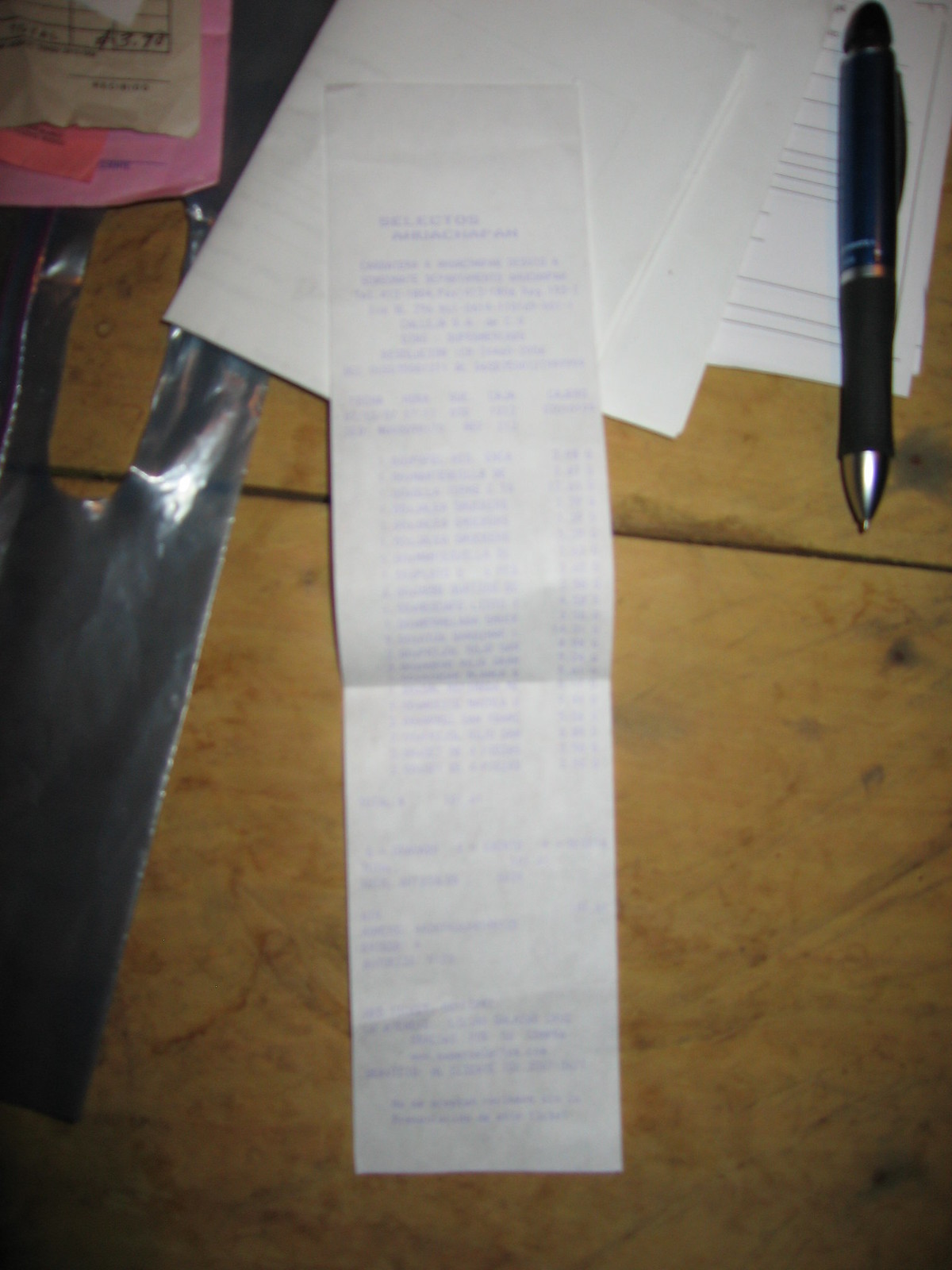The image presents a vertically rectangular frame of a very dimly lit interior, casting a subdued ambiance throughout the scene. At the bottom, we're gazing down onto a counter or desk surface that is predominantly tan-colored, adorned with darker tan to orange marbling patterns. Dominating the left side is a slightly angled, silver object, most likely a plastic bag, adding a touch of metallic sheen amid the muted tones.

In the upper section of the frame lies a stack of papers, the bottom edges of which fan out delicately to the right, indicating a casual placement. To the right, aligned vertically, is a black pen with a sleek silver tip, pointed downward as if recently put down after a writing session. Crowning the center of the composition is a lengthy receipt with blue print, its text blurred or faded to the point of being unreadable, suggesting it has been there for a while or the lighting isn't conducive for clarity. The interplay of these objects creates a snapshot of casual clutter, narrating a moment of paused activity in a dim, tranquil setting.